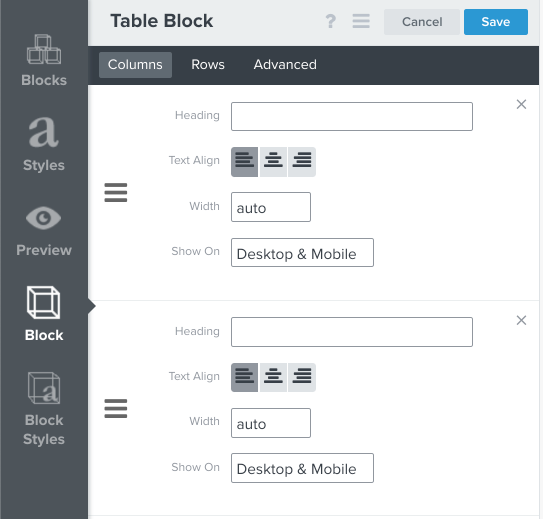**Detailed Image Description:**

The image features a user interface layout with a light blue border at the top. Centralized within this border, the bold black text reads "Table Block". Adjacent to this heading, there is a question mark icon and a hamburger menu icon. Just below this, there are two buttons: a gray button labeled "Cancel" and a light blue button labeled "Save".

On the left side of the image, there is a vertical dark gray column. This column contains the following labels, each in a descending order: "Blocks," "Styles," "Preview," "Block," and "Block Styles."

At the top of the main content area, there’s another bold heading that says "Heading". Accompanying this heading is a text input box, which has a small "X" icon on its right side. Below this text box, the label "Text Align" is displayed alongside three alignment icons (typically left, center, and right alignment). Following this section, there’s a heading labeled "Width" next to a text box displaying the word "Auto". Further down, there is another heading "Show On" with a text box beside it that reads "Desktop and Mobile."

This structure repeats once more in the image. There is another "Heading" label with an empty text input box. Below this, the "Text Align" label appears again with the same three alignment icons. The "Width" section follows with a text box displaying "Auto". Lastly, the "Show On" section is repeated, featuring a text box that again reads "Desktop and Mobile."